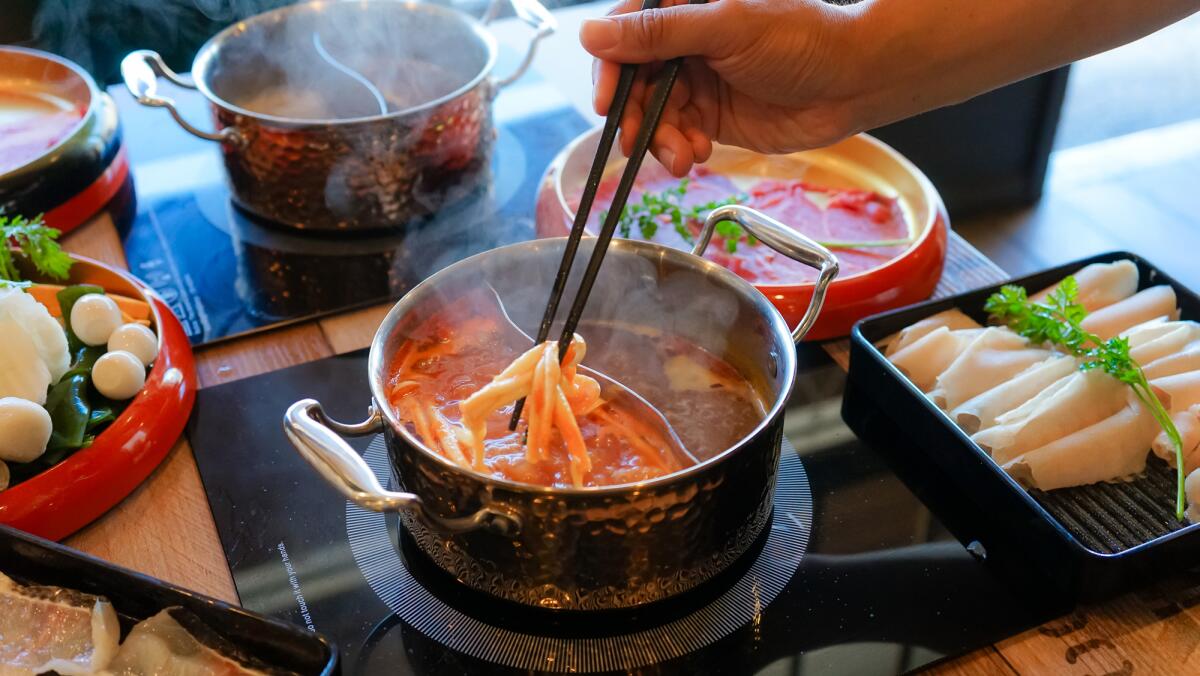The horizontally rectangular, full-color photograph captures a variety of dishes being prepared indoors during daytime, with natural light streaming in from a window. Central to the image is a pot with two handles, filled with a reddish-orange sauce. Emerging from this pot are noodles being lifted by a right hand holding a pair of chopsticks. The pot features a divider, separating a thicker sauce on one side from a thinner side. Adjacent to this central pot, another two-handled pot in the background is visible, also with dividers and steaming, but its contents remain obscured.

To the lower right corner, a black tray holds what appears to be rolled-up white slices, likely ham or turkey, garnished with a sprig of parsley. Nearby, another red bowl contains a liquid substance, while to the upper left, another red bowl holds items that possibly include greenery, such as peppers and eggs, or even a salad with round elements that could be either eggs or cheese balls. Additionally, a red plate with indistinct food is observed behind the main pot.

On the left, another red-trimmed plate is visible with food that is hard to identify, potentially hinting at Japanese cuisine. Despite the variety of dishes, the focus remains on the act of cooking with chopsticks and the array of components adding to the rich complexity and texture of the photograph. No people are fully visible in the image, emphasizing the food and culinary action.